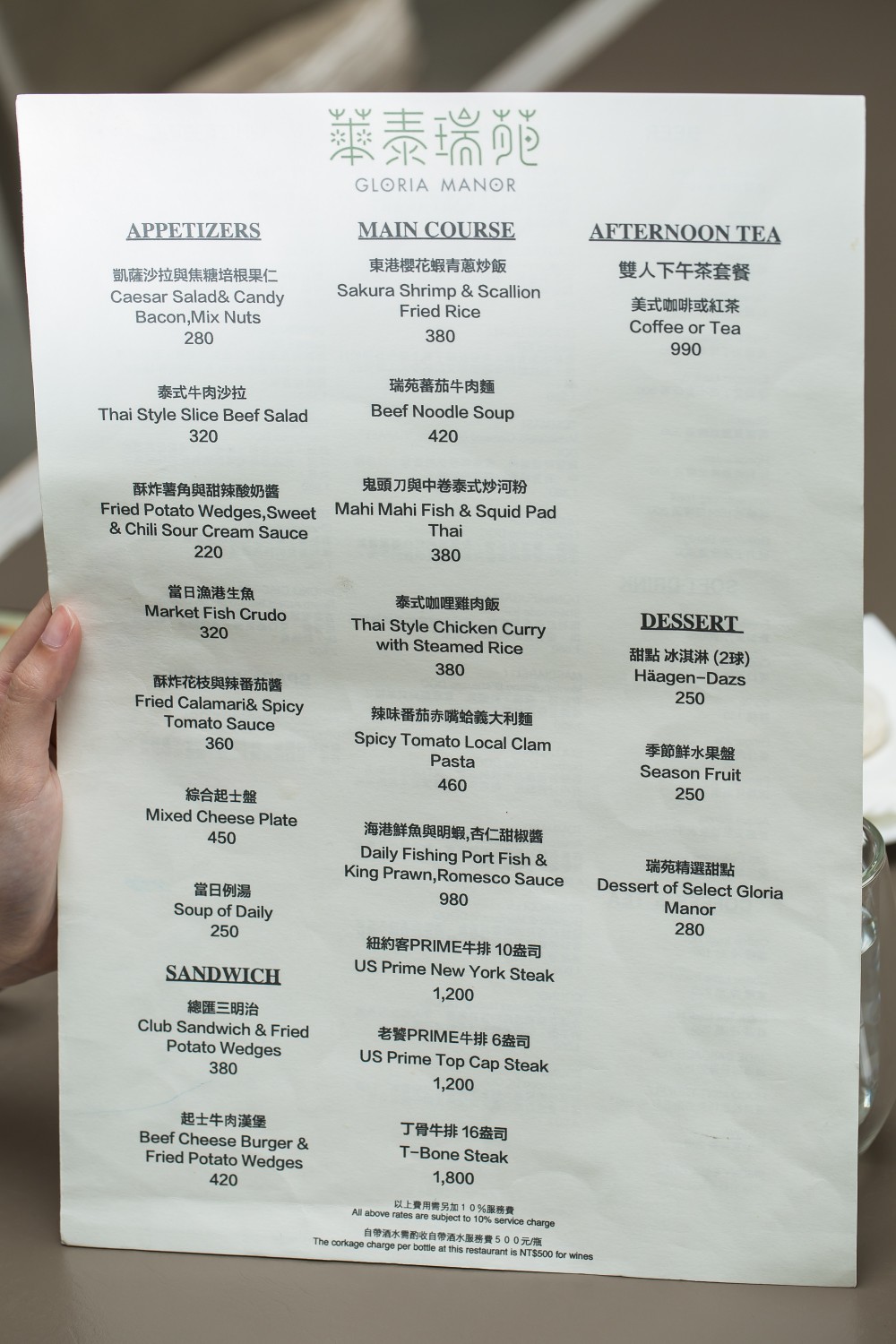In the image, a hand holds up a single white sheet of paper that serves as a menu at a restaurant. The background is blurred but suggests the presence of a tan table. The menu is gripped on the left side by a thumb, revealing no fingernail polish, with the remaining fingers obscured behind the paper. 

At the top of the menu, green symbols are displayed, followed by the name "Gloria Manor." The menu is divided into sections such as appetizers, main courses, afternoon tea, and dessert. Items are listed first in Chinese characters, accompanied by their English translations. The prices suggest a different currency, possibly Japanese yen, as indicated by items such as "Thai Style Sliced Beef Salad" priced at $3.20 and "T-Bone Steak" at $1,800, making it clear that the values are not in US dollars.